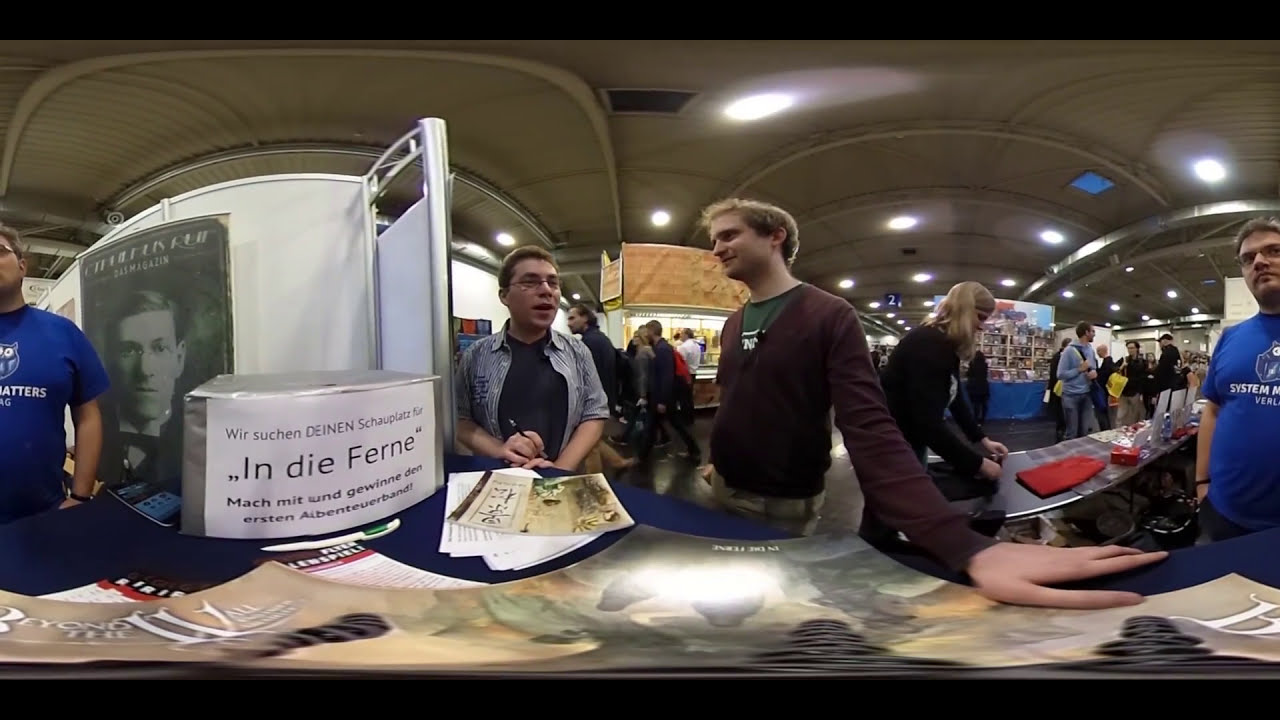This image captures a bustling convention or trade show set up in an indoor arena or gymnasium with dark flooring and a notable white ceiling adorned with curved lines and lights. Blue tablecloths adorn the various booths, where people are seen milling about, engaging with exhibitors. A striking feature of the photograph is the significant lens distortion, which makes spatial dimensions challenging to discern and notably exaggerates certain elements, such as a person's hand in the foreground.

In the immediate foreground, scattered pamphlets or magazines are visible on a desk. A man in a purple shirt, his hand disproportionately enlarged due to the lens effect, converses with another individual wearing a black T-shirt with sleeves rolled up. Adding to the ambiance, there's a prominent, partially readable sign in what seems to be German. The sign includes the word "Indiefern" alongside other smaller, illegible text. 

The intriguing lens distortion also creates a mirror-like effect, portraying the same person in a blue shirt with an owl graphic on both the far right and left sides of the image. Throughout the scene, multiple figures in varied attire, such as striped shirts and tan pants, are engaged with the displays and each other, making the scene rich with interaction and activity. A picture of a man in a bow tie on a white wall further anchors the space, suggesting a focal point or notable individual associated with the event.